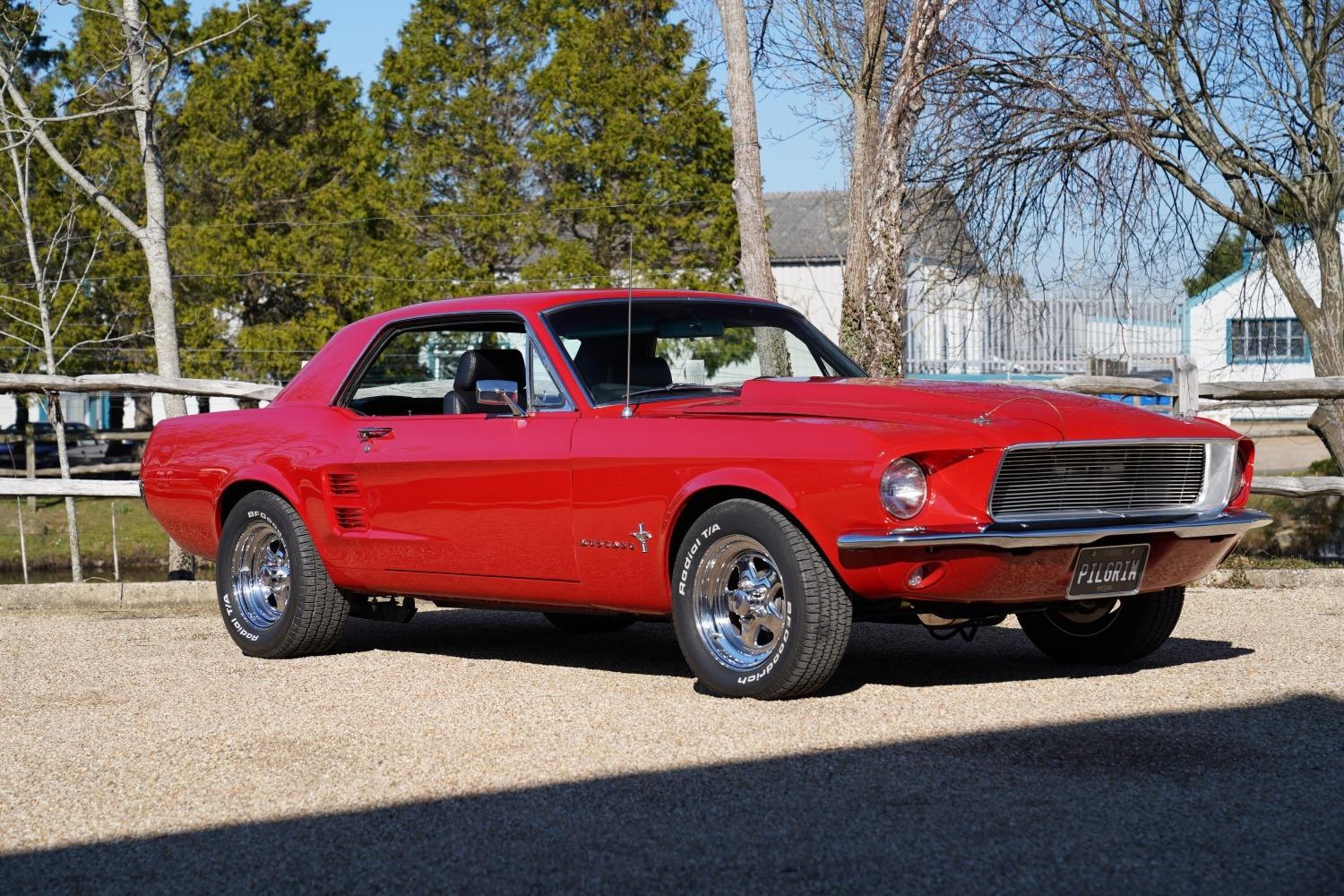The image features a restored, cherry red 1967 Ford Mustang, glowing under the sunlight with its pristine paint job. The Mustang's aggressive, yet classic body style boasts chrome wheels that appear to be original factory style, a black interior, and distinctive features including a hood cowl and hood latches tethered by a braided metal line extending into the front grille. Notably absent is the iconic Mustang logo, replaced by a black front license plate that reads "Pilgrim" in white letters. Set against a backdrop of green leaf trees and bare-branched trees, the scene also includes a house with white siding and blue trim, and a wooden timber railing. The car casts a shadow on the concrete where it's parked, adding depth to the vibrant outdoor setting.